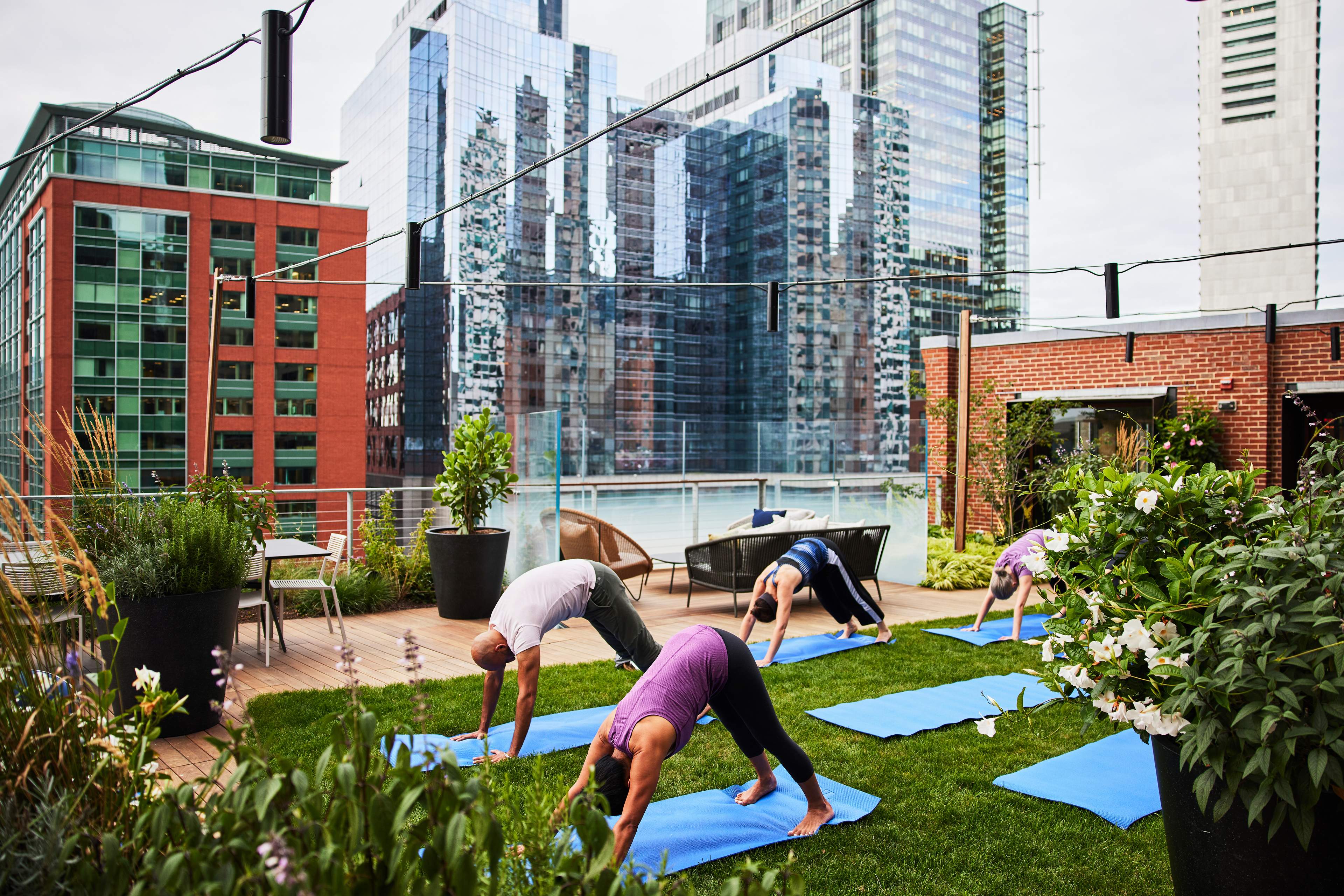This photograph captures a serene yoga session taking place on a rooftop in a bustling cityscape. The scene features four individuals, three women and one man, practicing yoga on a large grass-like mat area, each with a blue yoga mat. They are all in a downward dog position, with hands and feet grounded firmly and their bodies forming upside-down V shapes. Surrounding them are numerous large potted plants, adding a touch of greenery to the urban setting. The rooftop setup includes a brownish brick or wooden deck area and part of a brick facade from the hosting building is visible behind them. The background reveals a variety of high-rise buildings, some with reflective, mirror-like surfaces and others with red brick exteriors accented by green-tinted windows and window boxes, indicating residential apartments. The combination of the natural elements on the rooftop and the towering buildings creates a juxtaposition of tranquility amidst urban density.